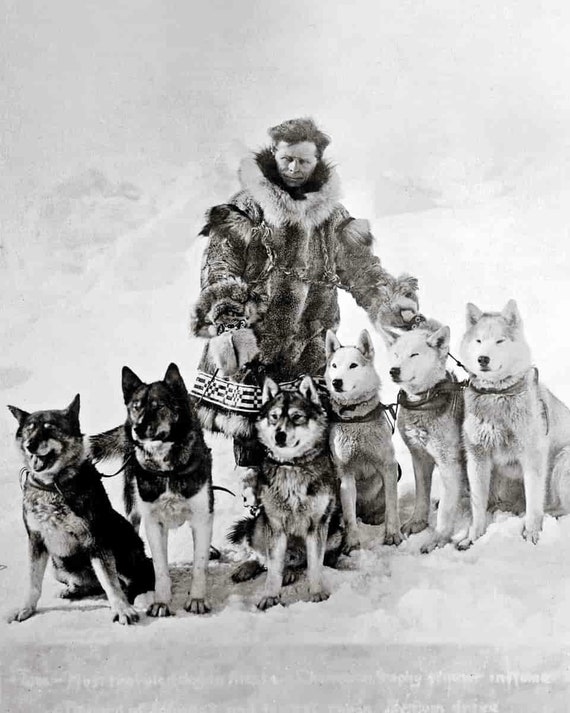This vintage black-and-white photograph captures a moment likely set in the Arctic or Alaska, featuring a solitary man standing amidst a vast expanse of snow. He is clad in a heavy fur coat, possibly made of animal fur, and wears thick, heavy gloves suitable for the freezing conditions. The man, who appears to be in his 30s with short hair, gazes into the camera with a look of determination. In front of him are six sled dogs, all secured with leashes around their collars. The dogs, resembling a mix of Huskies and perhaps other breeds common to sled racing, are arranged from left to right. Three of the dogs have darker fur, while the other three are lighter, almost white. The background is a stark, snow-covered landscape, creating a white-out effect that isolates the subjects in a beautiful yet harsh environment. The bottom of the photograph bears some barely readable white text, hinting that this image might have been featured in a magazine. The overall photograph exudes a sense of adventure and resilience, typical of dog sled racing scenes.